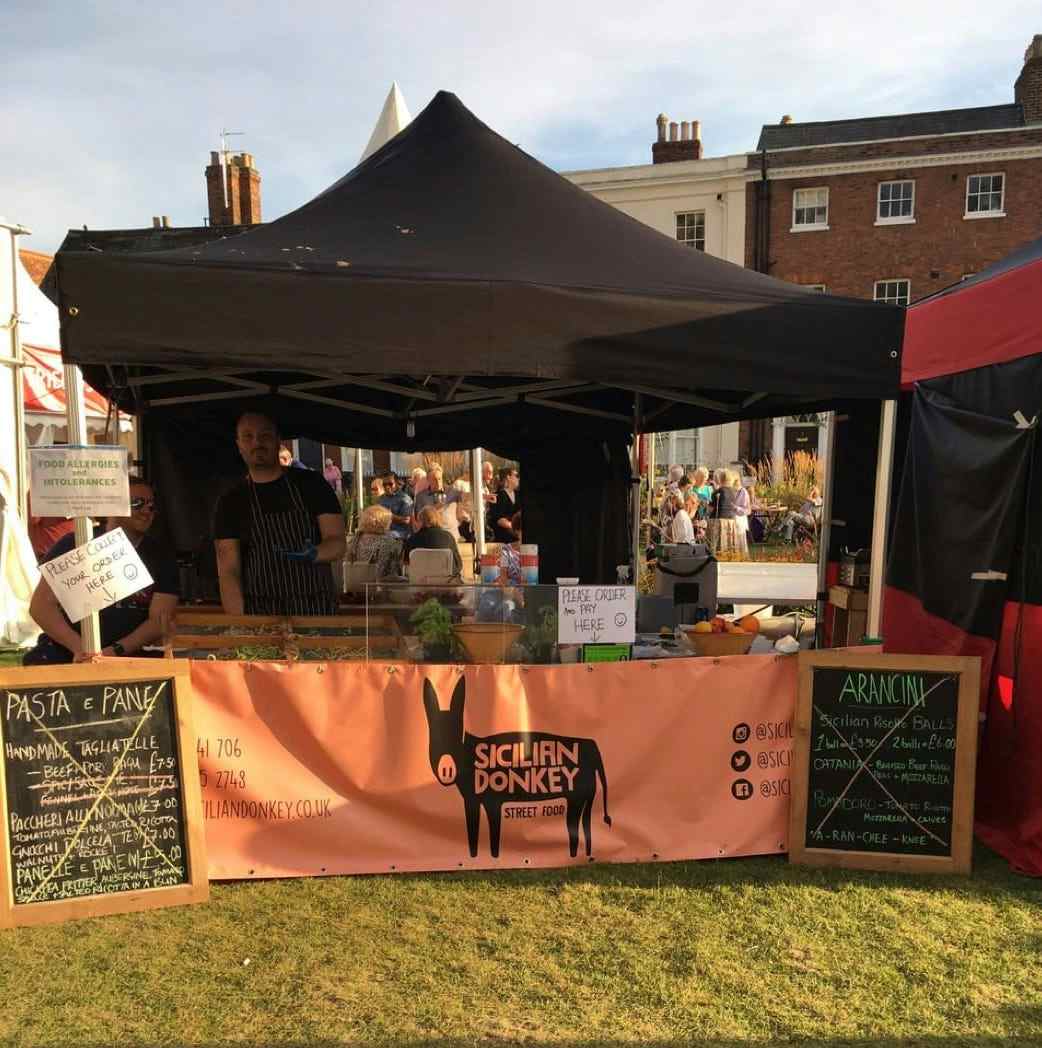In this vibrant daytime photograph of a street vendor’s booth at a bustling farmer's market, the setup under a brownish-black, tent-shaped canopy stands out against a backdrop of historic brick and white buildings. The bright blue sky, adorned with light clouds, adds to the inviting atmosphere. Central to the image, a distinctive orange banner with a black outline of a donkey and the words "Sicilian Donkey Street Food" catches the eye. This booth, placed on a lush grass surface, features two short chalkboards on either side, framed in blonde wood and listing menu items like "pasta e pane" and "arancini" in chalk. Inside the tent, two vendors attend to their stand, one donning a black shirt paired with a black and white striped apron. The stand itself is adorned with fresh oranges and potted plants, enhancing its charming, homegrown appeal. The presence of other canopies and a crowd hints at the lively market scene, making it a quintessential snapshot of community life.